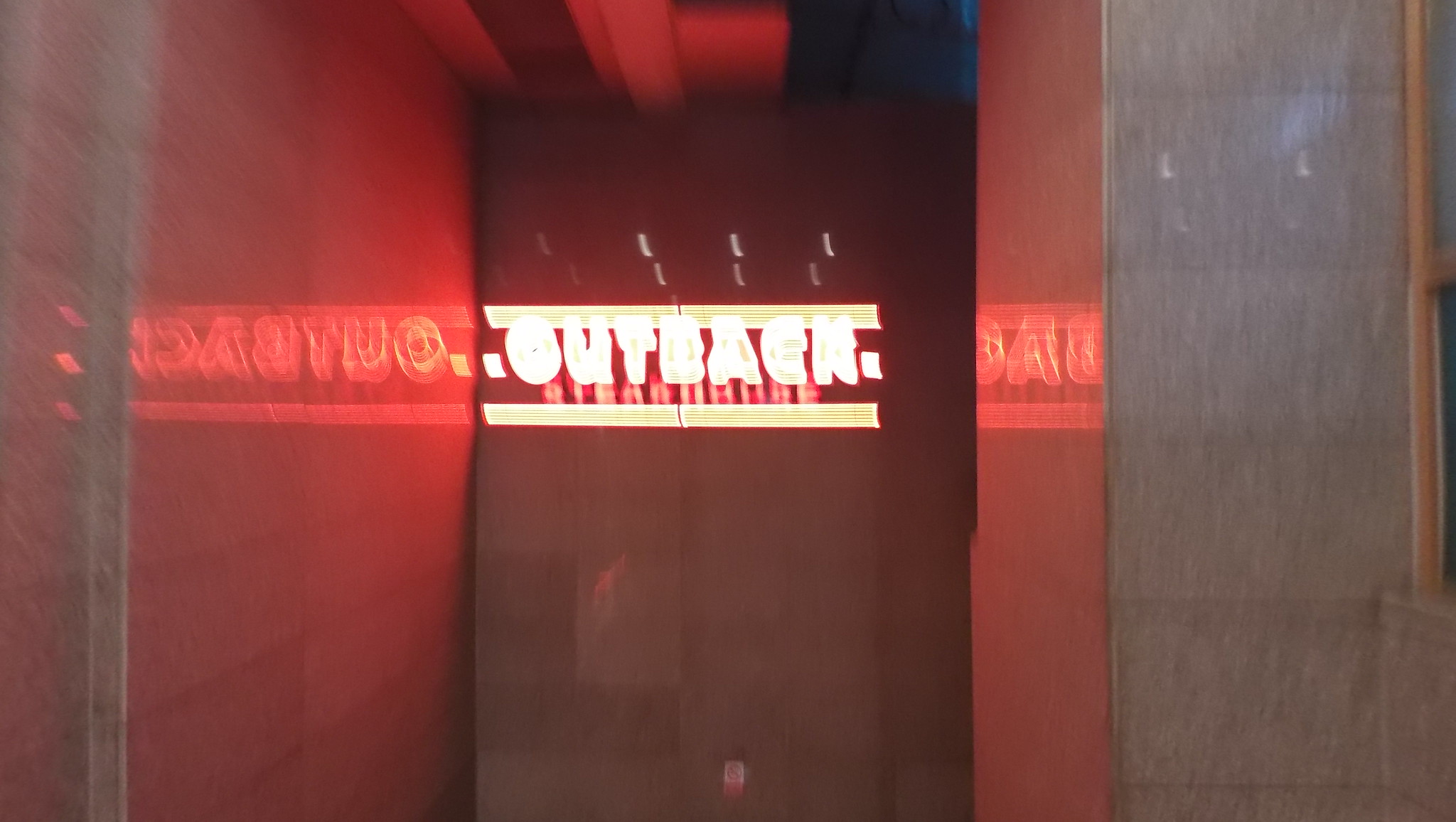In this blurred photograph, the focal point is an Outback Steakhouse sign. The image is unclear, making it challenging to discern precise details. The primary area shows a section of a wall painted in a gradient of gray tones transitioning into red. In the center, the Outback Steakhouse sign is prominently displayed. The sign features bold, white lettering with "OUTBACK" written in all capital letters, flanked by a line above and below the text. Below "OUTBACK," the word "Steakhouse" appears in smaller red letters, though it is difficult to make out clearly due to the blurriness.

The right side of the Outback sign seems to overlap into a red section of the background, creating a mirrored, backward effect of the text, which is also visible on the left side to a lesser extent. Additionally, there is a noticeable gray metal pole on the left-hand side of the image, contributing to the industrial ambiance. The photo's overall context suggests it might be taken in a hallway or entrance area, but the blur makes it hard to confirm this definitively.